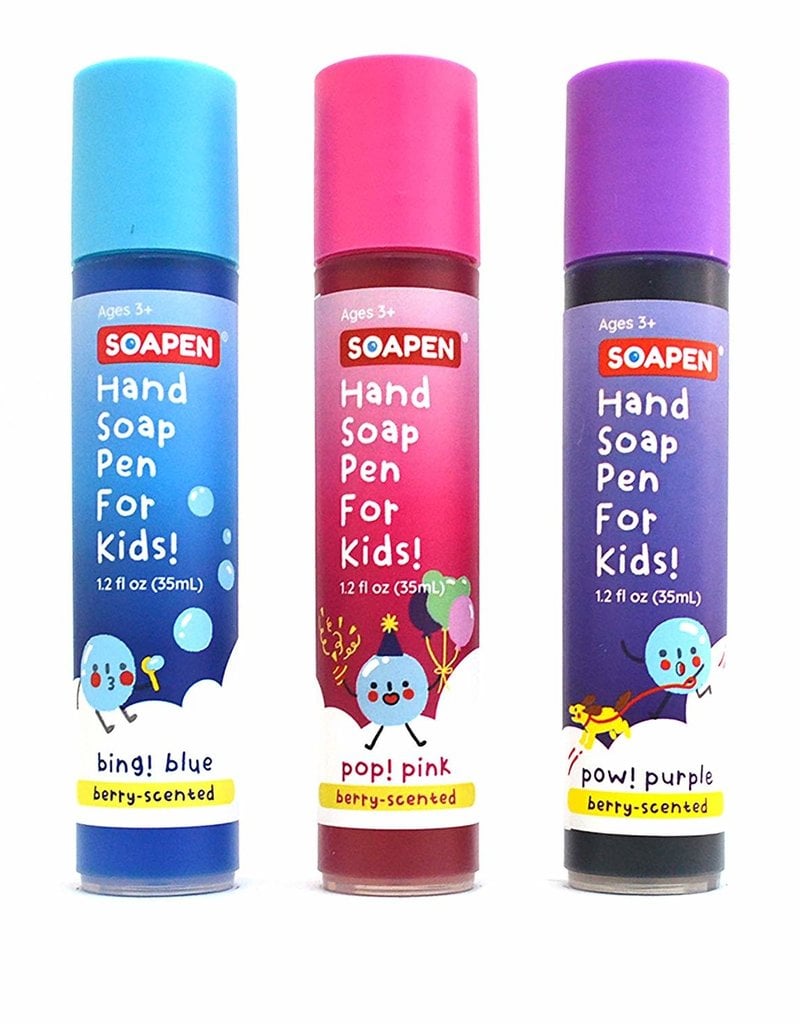This portrait-oriented color photograph is a product image featuring three vertical vials of hand soap for kids, set against a solid white background, giving the illusion that they are floating. Each tall, cylindrical tube has a cap and is partially transparent, preventing any visibility of the product inside. 

From left to right, the bottles are colored blue, pink, and purple. Each bottle has a consistent label design with slight variations in text and color cues: the blue bottle is labeled "Bing Blue, Berry Scented," the pink bottle is labeled "Pop Pink, Berry Scented," and the purple bottle is labeled "Pow Purple, Berry Scented." At the top of each label, the text reads "Hand Soap Pen for Kids," with a red horizontal bar logo above it stating "Soap Pen" in white text. 

Beneath the main text on each label is a yellow text box that reiterates the "Berry Scented" description. Each label features a line-art illustration of a circular blue character with round pink cheeks, displaying different expressions. This whimsical design element enhances the kid-friendly appeal of the product. The overall style of the image is realistic product photography, ideal for use in advertisements.